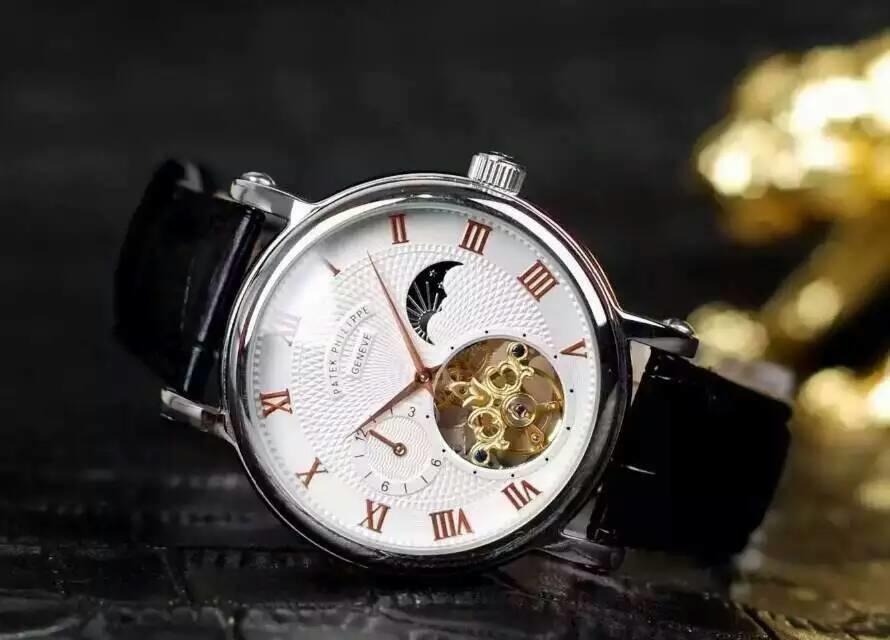This professional and highly detailed close-up photograph captures an exquisite Patek Philippe Genève wristwatch. The watch is positioned on a textured dark leather surface, accentuating its luxury. The background is dark, featuring blurred, golden lights in the upper right corner, possibly from string lights, adding a subtle glow. The focus is sharply on the watch, emphasizing its craftsmanship.

The watch boasts a black leather strap, visible on either side of the watch face, which curves elegantly behind it. The body of the watch is crafted from shiny silver chrome, enhancing its sophisticated look. The face of the watch is cream-colored with a finely textured surface and features bronze Roman numerals around its perimeter. 

Highlighted in the design is an exposed section of golden gears, visible through a circular cutout on the right side of the watch face, providing a glimpse into the intricate mechanics of the timepiece. Additionally, there is a smaller dial displaying seconds, and an icon indicating night and day. A unique black umbrella shape is also present on the right side of the watch face. 

Overall, the photograph captures the luxurious and intricate details of this Patek Philippe Genève watch, conveying its value and elegance.